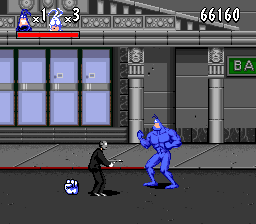In the screenshot of a computer game, a dramatic confrontation unfolds on a black roadway with a gray sidewalk. At the center of the scene, a towering male character dressed in blue armor—complete with blue gloves, integrated boots, and muscle-defining markings—faces off against a shorter, elderly man in a black suit who appears to be holding a gun and wearing a gray mask. Behind the man in black, there is an imposing, oversized hand in the shape of a fist on the ground. Both characters are situated in front of a building marked by two pillars and a roof, which appears to be a bank, as indicated by a green sign displaying the letters "BA." Above them, a scoreboard reveals the player’s score of 66,160 and a status bar with two icons: one showing the blue character with "1x" and the other a white character with "3x," likely indicating their lives or inventory.